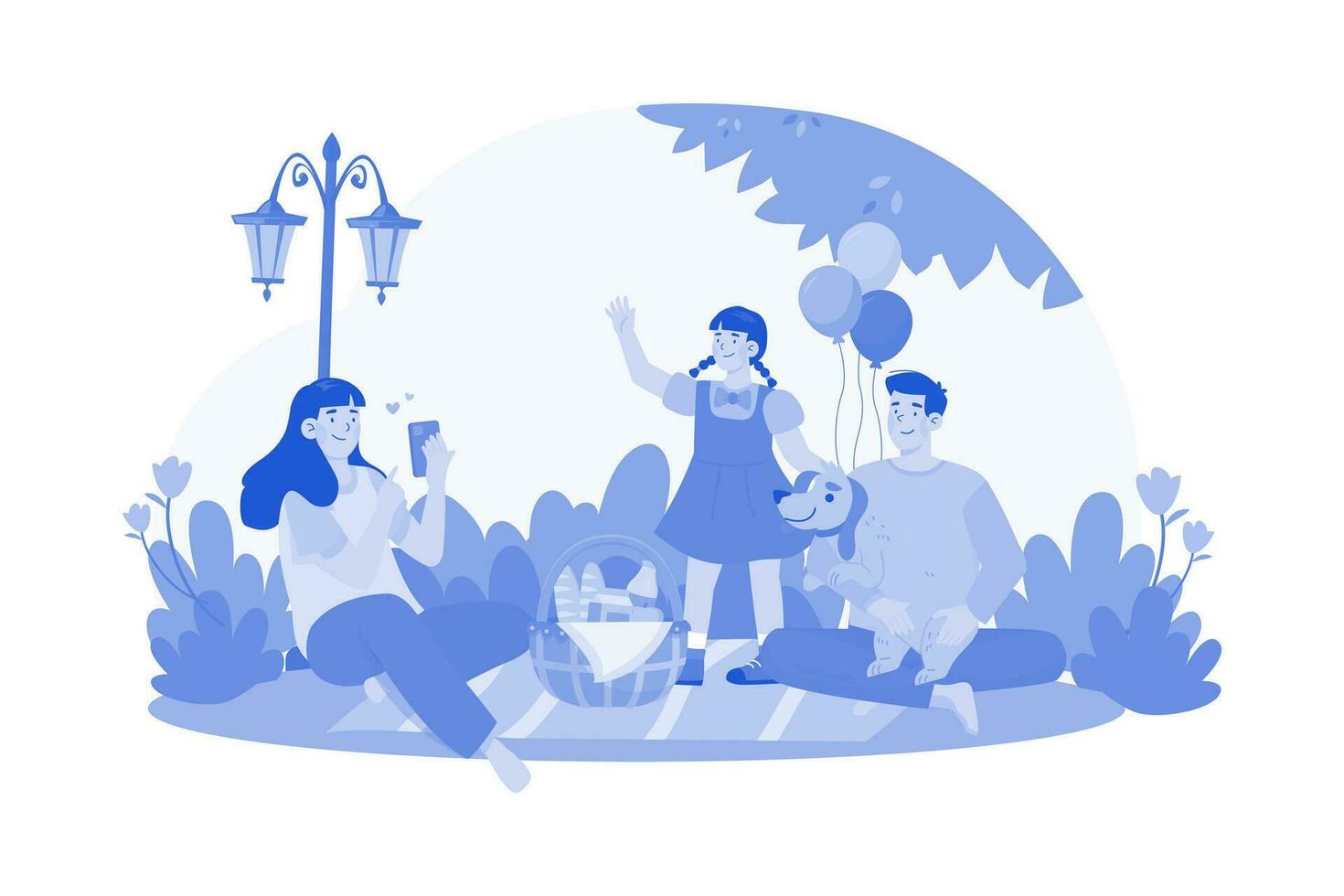The image is a monochromatic blue, cartoony illustration of a family enjoying a picnic. At the center bottom, a picnic blanket is spread out with a basket containing a baguette and a bottle. To the left of the blanket sits the mother, wearing dark pants and a white shirt. She has long, dark hair and is smiling while looking at a phone, appearing to take pictures. Behind her stands a lamppost with two lights, amidst various bushes and flowers. On the right side of the blanket, the father sits cross-legged, smiling, and holding a happy dog in his lap. He has dark hair, wears black pants, and a long-sleeved shirt. A little girl wearing a dress with pigtails and a bow tie stands between her parents, to the left of her father. She is waving with one hand while petting the dog with the other. Behind the father, three balloons float, adding a festive touch to the scene. The background features additional foliage, enhancing the outdoor, picnic atmosphere.